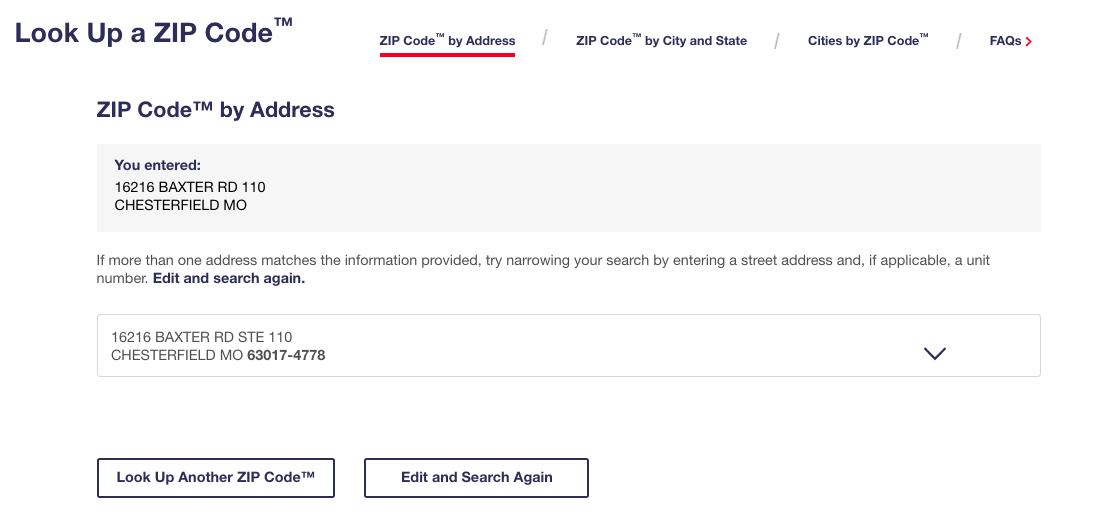The image is a screenshot from the USPS website, specifically from the "Look Up a ZIP Code" feature. In the top left corner, the text "Look Up a ZIP Code" is prominently displayed. A navigation bar spans across the top of the page with several buttons: "ZIP Code by Address," "ZIP Code by City and State," "Cities by ZIP Code," and "FAQs." The "ZIP Code by Address" button is highlighted with a red underline, indicating the current active selection.

On the left side of the screen, the section is labeled "ZIP Code by Address." The user has entered the address details, "16216 Baxter Road, STE 110, Chesterfield, MO." Beneath this, instructional text advises, "If more than one address matches the information provided, try narrowing your search by entering a street address and, if applicable, a unit number. Edit and search again."

A dropdown below displays the full matched address as "16216 Baxter Road, STE 110, Chesterfield, MO 63017-4778." At the bottom of the section, there are two buttons: "Look Up Another ZIP Code" and "Edit and Search Again," allowing the user to either perform a new search or refine their current search criteria.